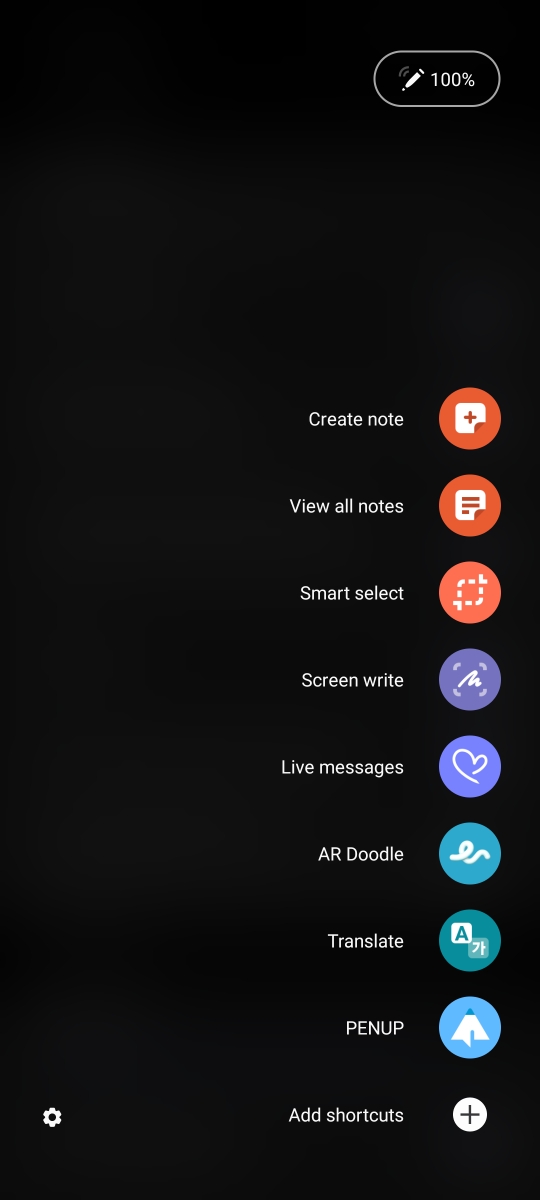The image depicts a detailed interface of a digital note-taking or editing application. On the left, there is a long black rectangular box. Adjacent to this, in the top right corner, is an elongated oval containing an icon of a white pen-like writing utensil, with "100%" displayed next to it.

Approximately four inches below this section, there is the option labeled "Create note" in white text. To its right, a red circular button houses a white square with a central plus symbol. Below this, the label "View all notes" appears with a corresponding red circle to the right, featuring a white square adorned with red lines.

Further down the interface, options are arranged as follows:
- "Smart select" which directly leads to "Screen write." The "Screen write" option is accompanied by a purple circle containing multiple white lines.
- "Live messages" represented by a purple circle with a white heart outline inside.
- "AR Doodle" depicted by a blue circle with a squiggly white line.

Continuing downward:
- "Translate" denoted by a teal circle with a white box containing the letter "A."
- "PENUP" written as P-E-N-U-P, accompanied by a blue circle featuring a white triangle.

The final option, "Add shortcuts," has a small white circle with a plus symbol to its right.